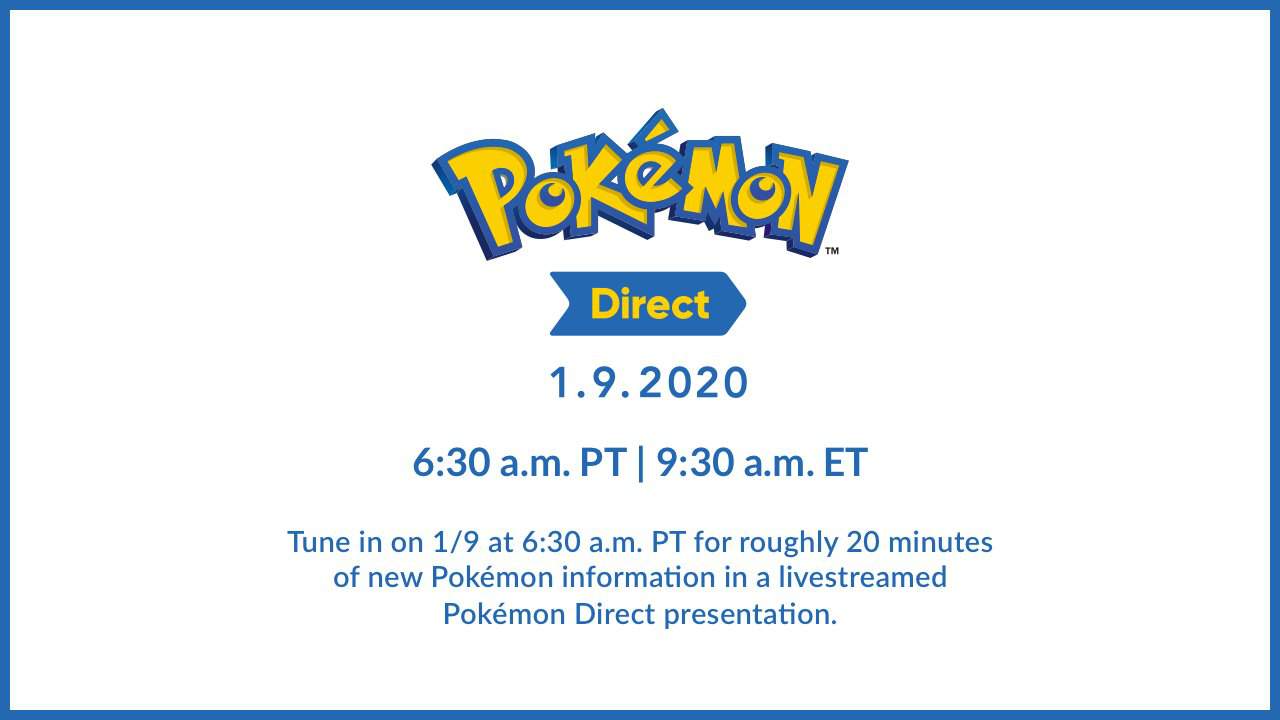The image is a rectangular banner in landscape orientation with a medium shade of blue outlining the perimeter. The background is white, and all the text is centered and presented in the same shade of blue. 

At the top of the rectangle is the iconic Pokémon logo, featuring the word "Pokémon" in bold yellow letters, outlined in blue and black. Directly beneath the logo is a blue, right-pointing arrow with the word "Direct" in yellow text inside it. 

Below the arrow, the date "1-9-2020" is prominently displayed, followed by the time "6:30 a.m. PT, 9:30 a.m. ET" on the next line. Slightly smaller text underneath this provides additional details: "Tune in on 1-9 at 6:30 a.m. PT for roughly 20 minutes of new Pokémon information in a live-streamed Pokémon Direct presentation."

The text and logo occupy the central third portion of the rectangle, ensuring that the detailed information is clearly visible and easily readable.